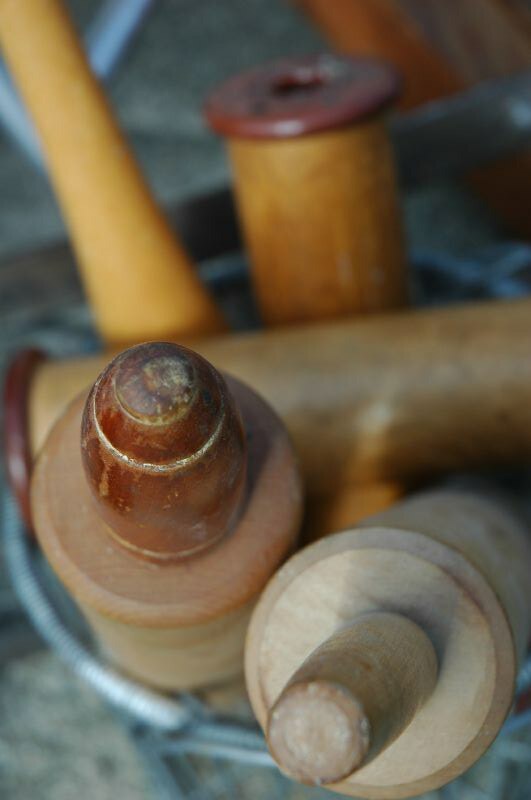In this photograph, although partially blurry, several rolling pins and other kitchen utensils are visible, placed in a wire container. The two nearest rolling pins are in focus and prominently feature. The rolling pin on the left has a lighter wooden body with darker, curved handles that include grooved details near the tips, indicating frequent use. The wooden rolling part is slightly thicker in the middle, perhaps showing a contrasting wear from the handles. The rolling pin next to it has a more uniform appearance, with the handles glazed and slightly thicker, creating a shiny finish. Further back, the rolling pins lose their clarity and do not exhibit detailed handles, with some appearing as plain cylinders. Additionally, other cylindrical objects, possibly pepper mills or bottles with darker tops, are discernible in the background, adding to the crowded and somewhat chaotic arrangement within the container. Despite the blur, the mix of textures and shades of wood draws attention to the utensils.